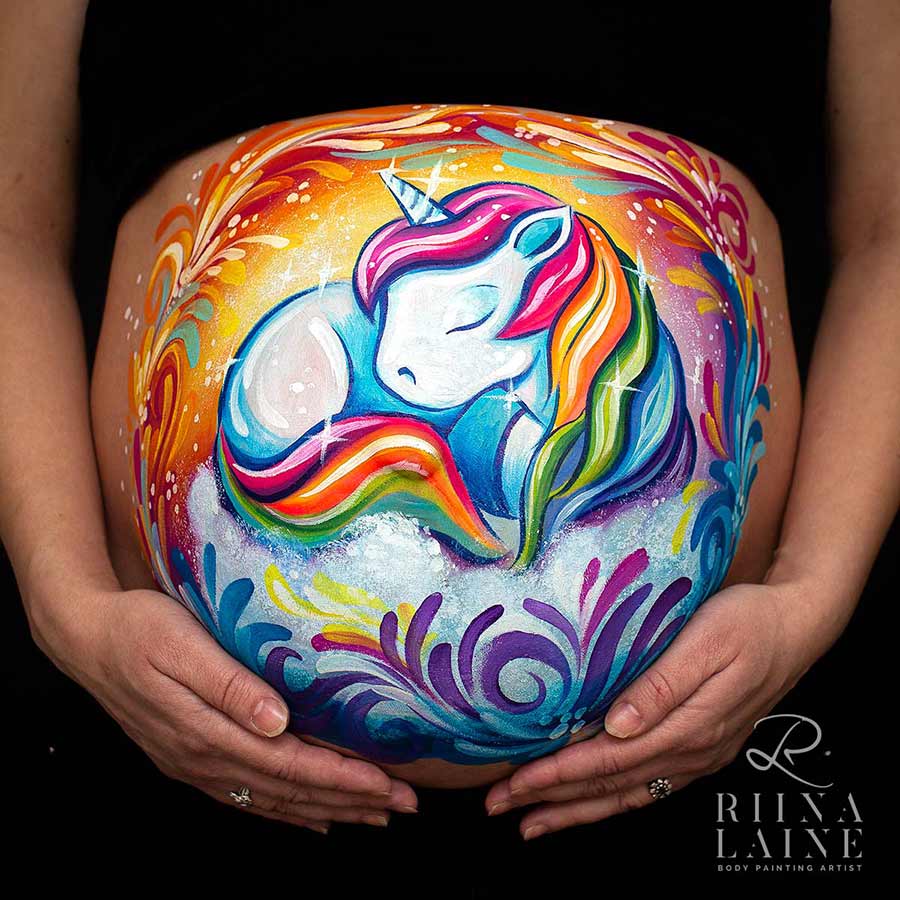This image is a large, square photograph capturing a pregnant woman's belly, with both of her hands gently cupped underneath it. Her belly is intricately painted with vibrant, rainbow colors. At the center of the artwork is a white unicorn, styled similarly to My Little Pony, lying down with its eyes closed. The unicorn features a rainbow mane that cascades down from its head.

Surrounding the unicorn are various colorful, leafy patterns – hues of purple and blue near the bottom part of the belly, where her hands support it, and red, orange, and yellow tones across the top. The woman is wearing a black shirt, which is pulled up to reveal her painted belly, and black pants. The shirt appears to be short-sleeved or sleeveless, as her bare arms are visible in the photo.

In the lower right corner of the image, there is a watermark with the name "Riina Laine," denoted in cursive, followed by the designation "Body Painting Artist." This artistic close-up beautifully showcases the unique body art and the tender moment of the woman embracing her pregnancy.